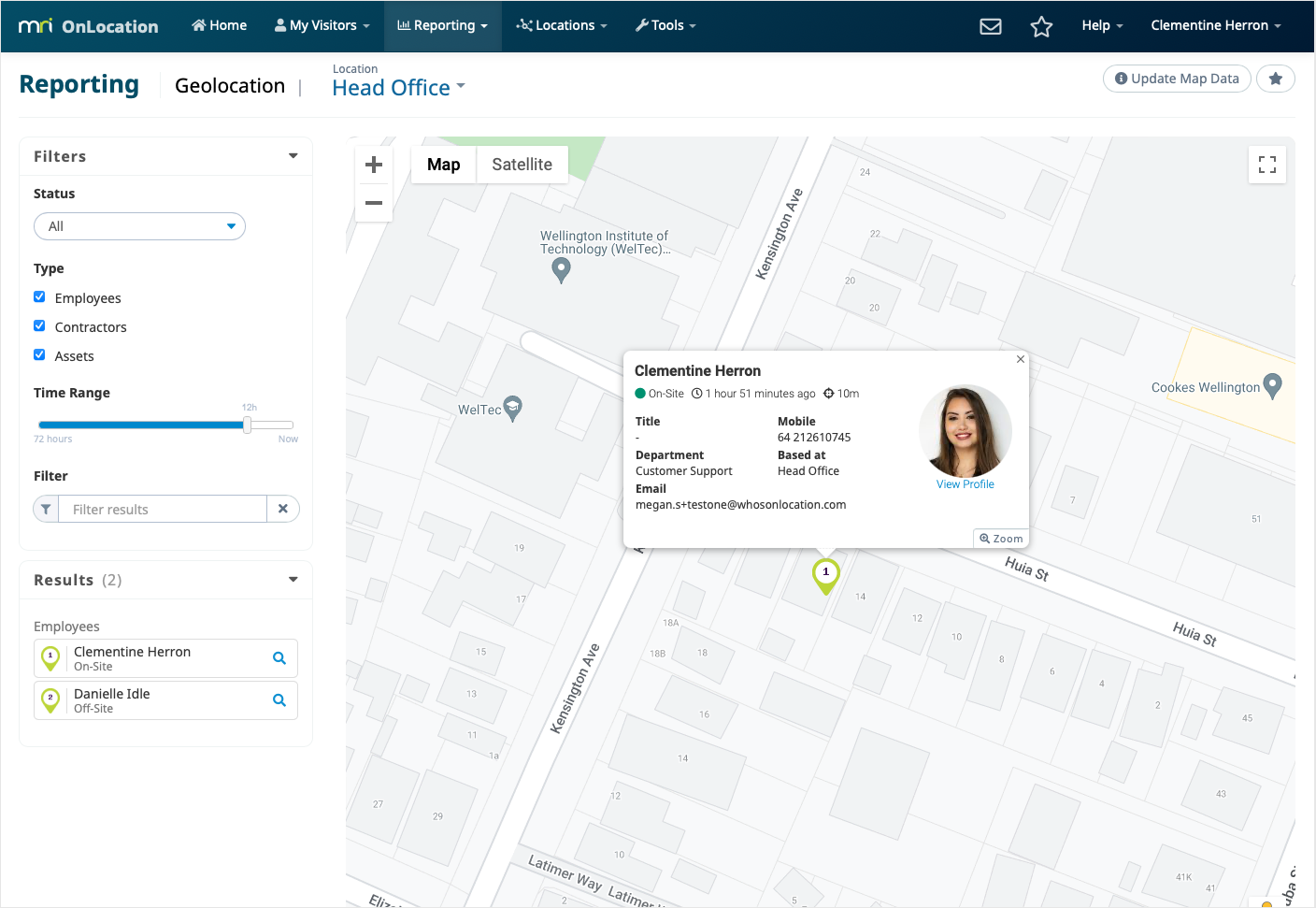Screenshot of the "MRI on Location" website, displaying the reporting page. At the top, the toolbar includes navigation options such as Home and My Visitors, with the reporting page currently selected. In the center of the screen, there is a detailed information card for Clementine Heron, featuring her profile picture. Clementine is a customer support representative, and her contact details, including email address and mobile phone number, are clearly visible. The backdrop of the information card is a satellite map, focusing on an area around the Wellington Institute of Technology.